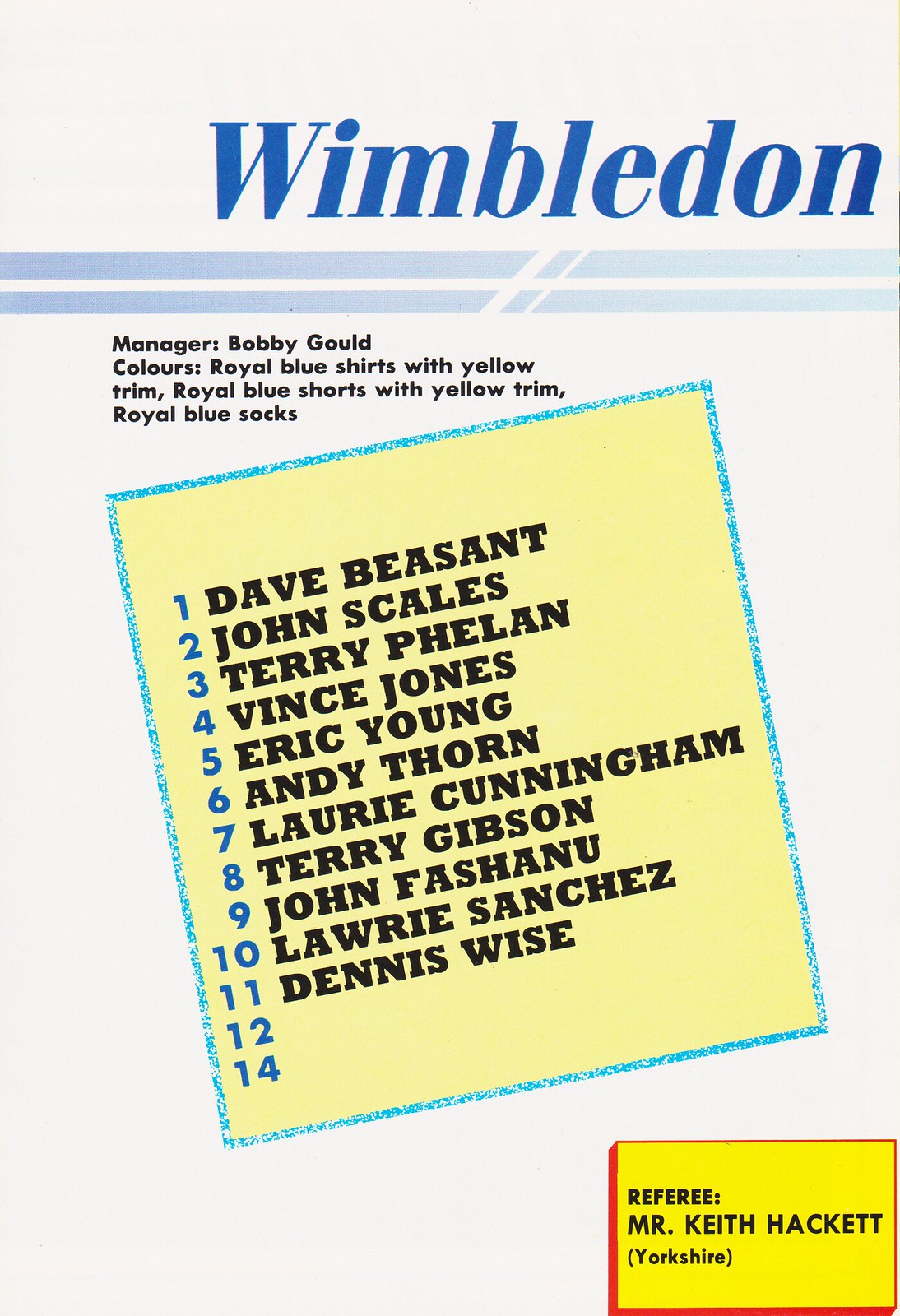The image depicts a detailed sports brochure featuring the Wimbledon football team. At the top, the word "Wimbledon" is prominently displayed in large, bold blue block letters, followed by two light blue lines. Just below this header, the manager is identified as Bobby Gould in black text. The team's colors are specified as royal blue shirts with yellow trim, royal blue shorts with yellow trim, and royal blue socks. 

In the center of the page, there is a blue-outlined square, tilted to the left with a yellow fill inside. Within the square, a list numbered from 1 to 14 appears, with numbers in blue and corresponding player names in black. The names listed are: Dave Besant, John Scales, Terry Phelan, Vince Jones, Eric Young, Andy Thorne, Laurie Cunningham, Terry Gibson, John Fasheneau, Laurie Sanchez, and Dennis Wise. 

At the bottom of the page, it mentions the referee, Mr. Keith Hackett, marked in yellow with red outlines. The brochure, potentially an advertisement for the football team rather than a tennis team, provides an overview of team members and relevant details in an organized layout.